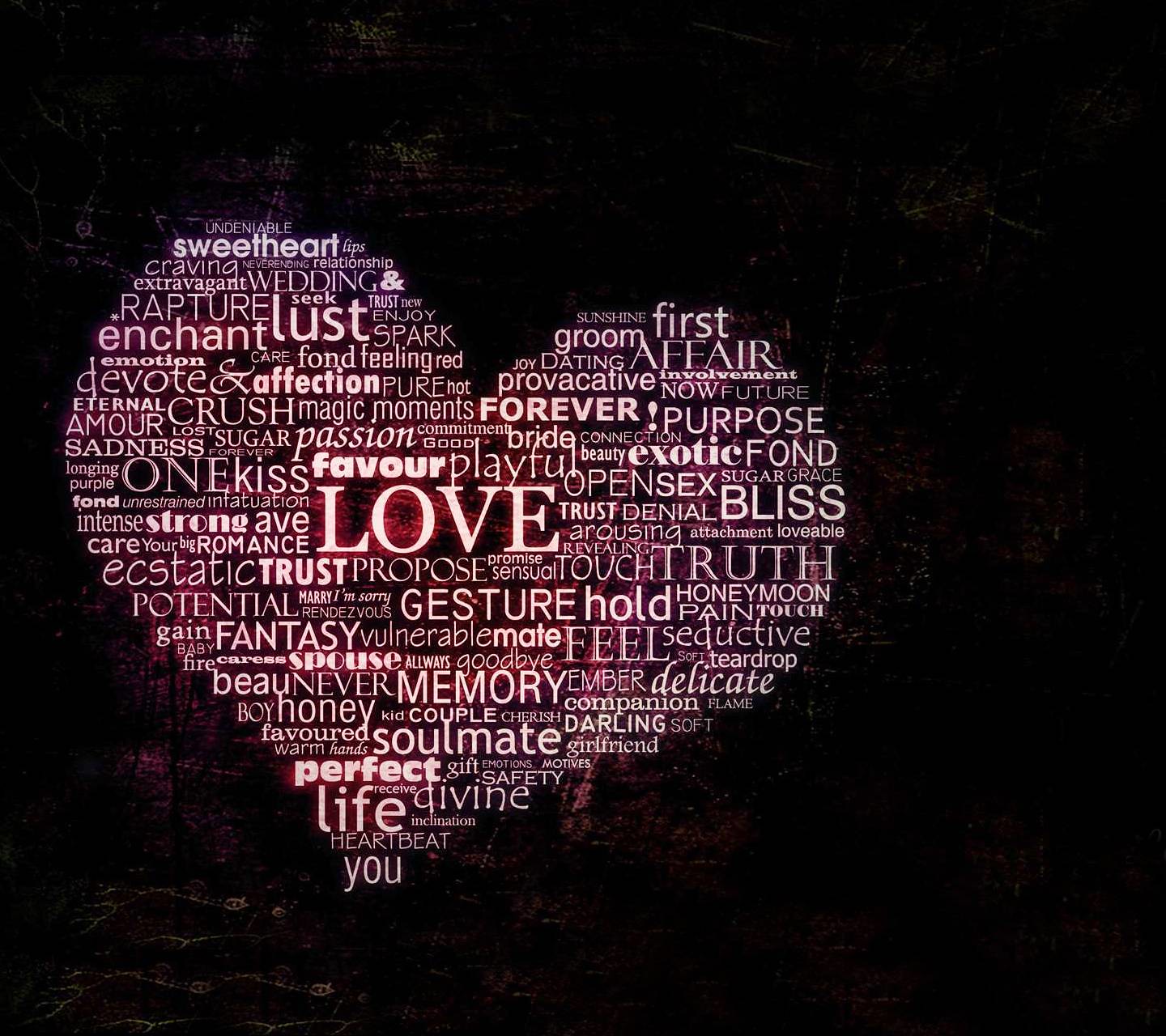The image is an artistic poster featuring a heart shape set against a dense black background sprinkled with subtle specks of pinkish and purplish hues. The heart itself is intricately composed of numerous words, all rendered in white and varying shades of pink, with differing fonts and sizes creating a rich textual tapestry. At the very center of the heart, the word "Love" stands out prominently as the largest element, surrounded by an array of intimate and romantic terms such as "Sweetheart," "Lust," "Rapture," "Feel," "Gesture," "Bliss," "Forever," "Affair," "Purpose," "Exotic," "Life," and "You." Additional words include "Craving," "Enchant," "Wedding," "Groom," "Dating," "Provocative," "Fond," "Trust," "Denial," "Undeniable," "Passion," "Thirst," "Soulmate," "Perfect," "Fantasy," "Propose," "Amor," "Eternal," "Heartbeat," "Open sex," and "Truth." The overall effect is a visually compelling collage that conveys themes of love, romance, and emotional connection, with the heart’s pink tones subtly contrasting against the dark background.